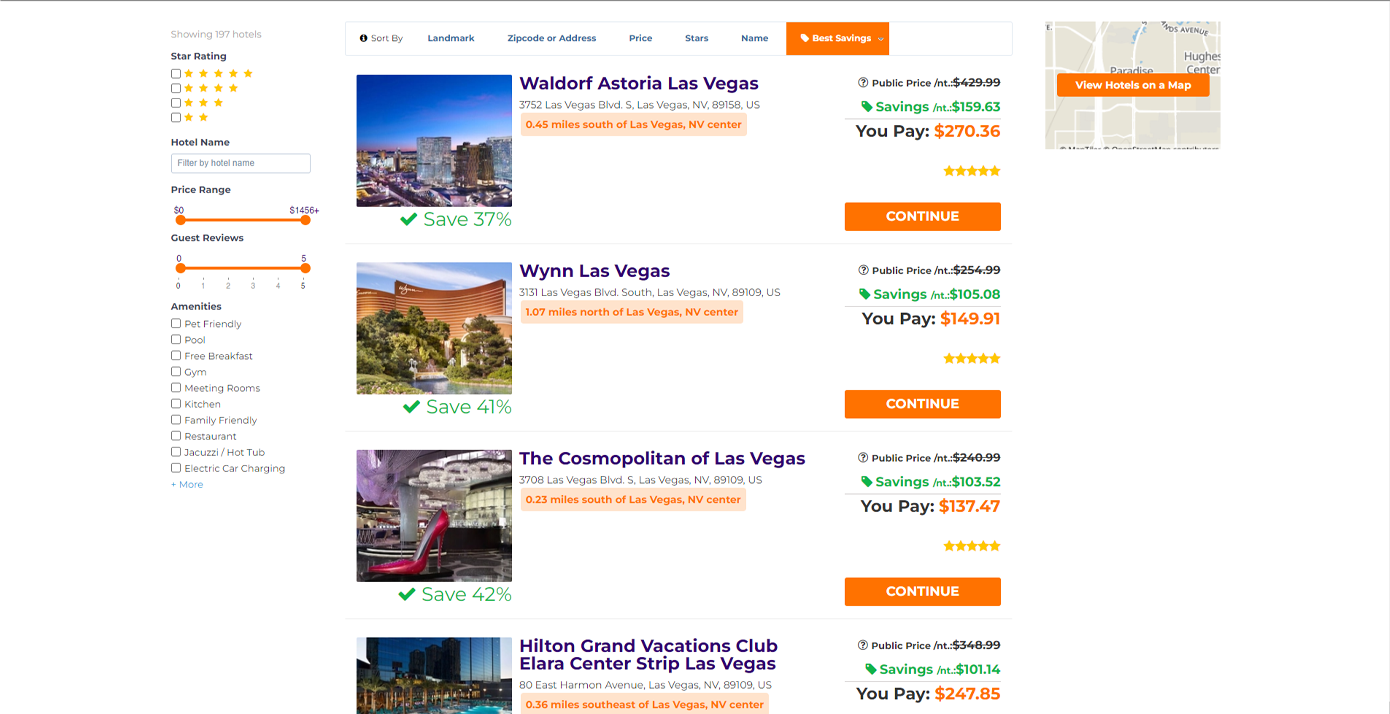### Detailed Caption for Hotel Comparison Web Page Screenshot

This image captures a screenshot of a webpage comparing hotels in Las Vegas. The interface is divided into sections with various filters and hotel options.

**Left Sidebar:**
- A list indicates "Showing 197 hotels".
- **Star Rating Filter:** Checkboxes for ratings from 5 to 2 stars.
- **Hotel Name Filter:** Allows users to filter by hotel names.
- **Price Range Slider:** Ranges from $0 to $1456+.
- **Guest Reviews:** Ranges from 0 to 5.
- **Amenities Filter:** A detailed list of amenities with checkboxes, such as free breakfast, pet-friendly options, and electric car charging stations, with a clickable “+ More” link.

**Main Content (Middle Two-Thirds):**
- **Sort By Dropdown Menu:** Options to sort by landmark, zip code or address, price, stars, name, with "Best Savings" highlighted in orange.

**Displayed Hotels:**

1. **Waldorf Astoria Las Vegas**
   - **Image Description:** A distant view of the hotel, amidst other buildings, in the evening with a dusky blue sky.
   - **Price:** $270.36 (Public price: $429.99)
   - **Savings:** $159.63, indicating save 37%.
   - **Rating:** Five stars.
   - **Address:** 3752 Las Vegas Boulevard South, Las Vegas, NV 89158, US. 0.45 miles south of Las Vegas Nevada Center.
   - **Action Button:** “Continue” in orange.

2. **Wynn Las Vegas**
   - **Image Description:** A curved golden building with "WYNN" in cursive, tall trees, and a water feature in front.
   - **Price:** $149.91
   - **Rating:** Five stars.
   - **Address:** 3131 Las Vegas Boulevard South, Las Vegas.
   - **Action Button:** “Continue” in orange.

3. **The Cosmopolitan of Las Vegas**
   - **Image Description:** Interior view featuring an oversized red high-heeled shoe, high-class bar with crystal lighting, purple lavender netting, shiny floor, and stage-like pillar.
   - **Price:** $137.47
   - **Rating:** Five stars.
   - **Address:** 3708 Las Vegas Boulevard South, Las Vegas.
   - **Action Button:** “Continue” in orange.

4. **Hilton Grand Vacations Club E-L-A-R-A Center Strip Las Vegas**
   - **Image Description:** A glass building with numerous windows, palm trees, and a pool in front.
   - **Price:** $247.85
   - **Address:** 80 East Harmon Avenue, Las Vegas.

The fourth hotel’s information appears partially cut off in the screenshot.

This screenshot provides a comprehensive overview of hotel choices in Las Vegas, featuring price comparisons, ratings, and visually descriptive images to aid in selecting the most suitable accommodation.